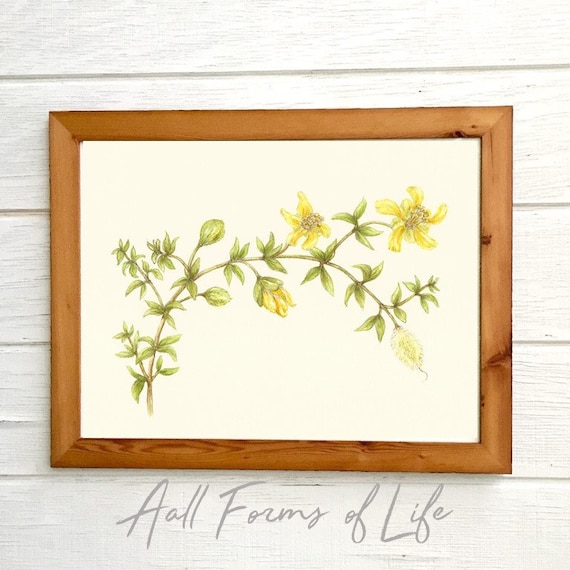The image features a striking framed print mounted on a gray-toned wall with visible wood grain and five wooden panels. The frame surrounding the print is made of medium brown wood, adorned with darker knots and striations. Inside the frame, the print presents a white or cream-colored background showcasing a gracefully curved branch. The branch starts from the bottom left and arches toward the upper right. Adorned with lush green leaves, the branch exhibits various stages of yellow flowers. Near the bottom, the flowers are beginning to bud, while towards the middle and top, the flowers are fully bloomed with wide-open petals. A few flowers and buds show signs of aging, hinting at a complete life cycle. Below the elegant display, in gray cursive script, is the phrase "AALL forms of life," emphasizing the diversity and stages of life depicted in the artwork.